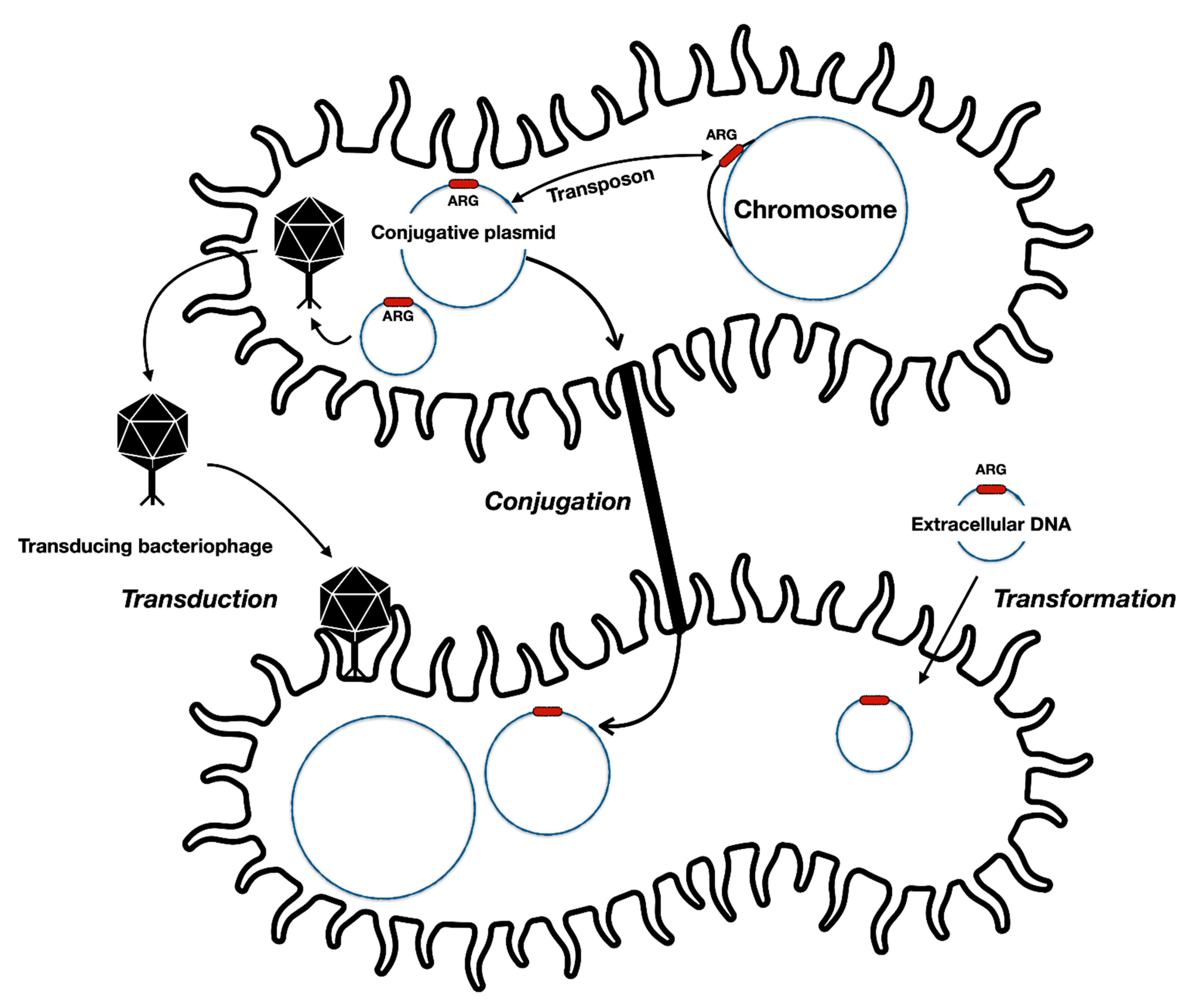The image is a detailed black and white illustration with red highlights, depicting the biological processes of transduction, conjugation, and transformation in bacteriophages. The top portion of the image illustrates a prokaryotic cell or possibly a mitochondrion, featuring a labeled chromosome and a conjugative plasmid. Arrows indicate the flow of genetic material, showing a plasmid moving between cells via a process labeled conjugation. A transducing bacteriophage is depicted in the act of transferring genetic material, symbolizing transduction.

The lower part of the image continues this theme, showing another prokaryotic cell with labeled extracellular DNA bits in red, indicating transformation. The entire illustration meticulously demonstrates the steps and components involved in genetic material transfer among bacteria, emphasizing the role of chromosomes, plasmids, and bacteriophages. The repetitive use of terms such as 'chromosome,' 'conjugative plasmid,' 'transduction,' and 'extracellular DNA' underscores key elements of these biological processes.